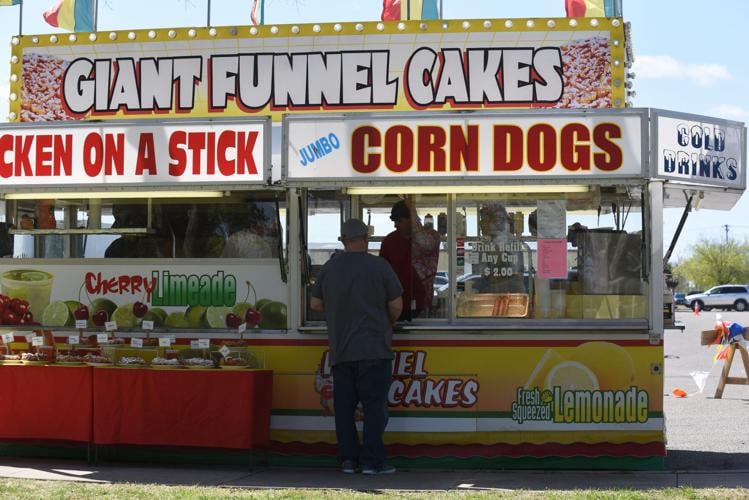Here's a detailed and cleaned-up caption for the image:

---

The vibrant sidewalk snack stand, adorned with multicolored lights around its perimeter, prominently displays the sign "Giant Funnel Cakes." Resembling the festive booths often found on a bustling boardwalk or at a lively fair, the stand is a visual feast with its striking yellow and red color scheme. Large, bold lettering advertises "Chicken on a Stick" and "Jumbo Corn Dogs," indicating the variety of comfort foods available. A cheerful man operates inside the stand while another stands outside, attending to curious customers. The stand also offers "Cherry Limeade," as stated on one of its signs. In front of the stand sits a table laden with an assortment of items, possibly pies, cakes, lemonade, and other cold drinks, ready for sale. A special promotion offers drink refills for $2 with the purchase of any drink cup. The stand itself stands approximately 25 feet long and 12 feet tall, making it a noticeable and inviting spot for passersby.